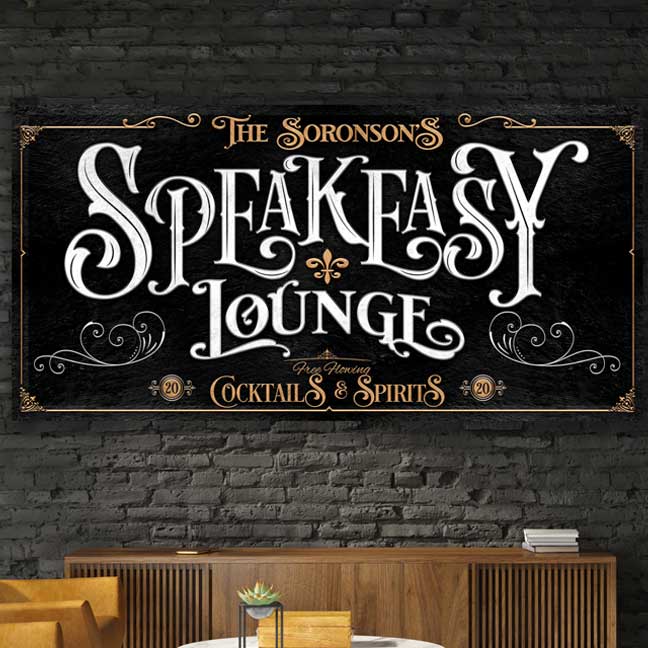This photograph captures the interior of a stylish lounge featuring a dark gray, monochrome brick wall adorned with an elegant sign. The rectangular sign boasts a black background, gold border with ornamental corners, and a center adorned with a fleur-de-lis. At the top, in smaller gold text, reads "The Sorensons," and beneath it, the bold white text proclaims "Speak Easy Lounge." Below, it states in matching gold letters, "Cocktails and Spirits" flanked by intricate filigree designs. Positioned against the wall, a modern tan Danish-style credenza holds three stacked white books at one end. In front of the credenza, a round white coffee table is adorned with a golden wooden box and a succulent plant in a black wrought iron stand. Flanking this setup are two mustard-colored side chairs, adding a pop of color to the sophisticated space.